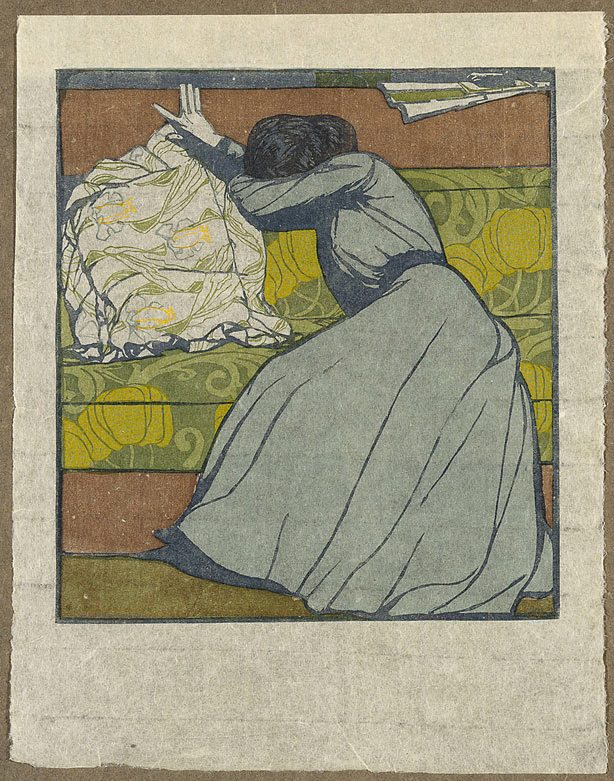The image is a detailed painting of a woman sitting on an intricately patterned sofa, which is olive green with yellow flowers or possibly pumpkins. The scene is bordered by a thin brown frame, and the background features a brown wall, lending a somewhat somber atmosphere to the setting. The woman, wearing a floor-length light grayish or bluish dress with a belt, is depicted in a moment of distress. She has dark hair and her head is bowed down between her raised arms. Her left side is more prominently visible, and she appears to be clutching the wall behind her with her right hand. A white blanket with a green and yellow pattern is casually tossed over the back of the sofa on the left side. The overall tone of the painting is dark, with the woman's posture and unseen face conveying a deep sense of sorrow. No other objects or people are present in the image, focusing the viewer's attention entirely on the woman's emotional display.